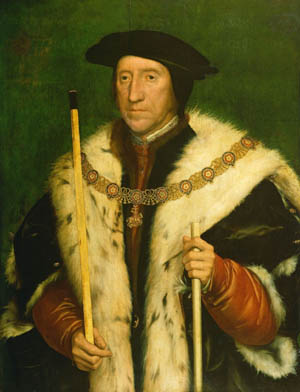This detailed, vertical rectangular image appears to be an old painting of a 17th-century man. The background is a dark green, enhancing the subject's stark appearance. The man, a white male with a long pointed nose and no visible eyebrows, stands confidently, his hair cascading to his collar. He dons a wide black hat, possibly a beret or cap with ear flaps, and wears a heavy coat with luxurious white fur lining that drapes around his shoulders and down his back. Beneath the coat, the red sleeves of another garment are visible, suggesting richness and warmth.

Prominently displayed across his chest is a chain of office with a medallion hanging down from it. The man’s eyes are dark, possibly black, adding to his stern, authoritative presence. In his right hand, he holds a short stick with a black top, and in his left, a longer one, resembling disassembled pool cues or walking sticks. This medley of distinctive features highlights his likely noble or royal status, depicted solemnly against the uniform dark green backdrop.